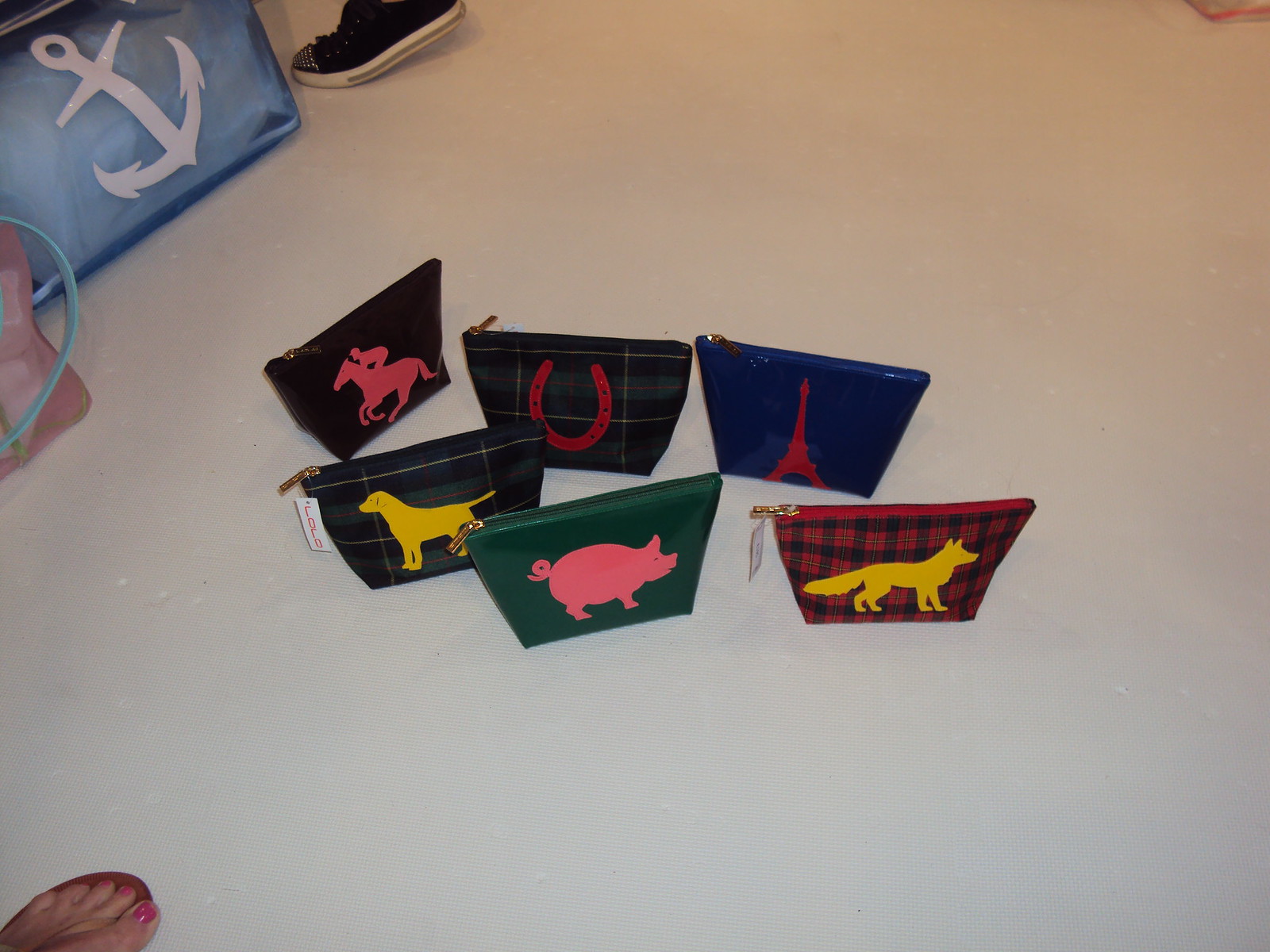This color photograph, taken from above, depicts a collection of six small coin purses arranged on a white floor. The floor extends as a large white area, possibly indicating a countertop or clean floor surface. In the bottom left corner, a person's foot in a sandal, with painted toenails, is visible, while the top left corner reveals a sneaker-clad foot, suggesting someone standing nearby. Each coin purse is distinct in design, though they share a similar size and silhouette-patterned fronts. In the top row, the leftmost purse features a red image of a jockey on a horse, followed by a purse with a red horseshoe, and a blue purse adorned with a red Eiffel Tower. The second row showcases a black purse with a yellow dog, a green purse with a pink pig, and a red and black checkered purse with an emblem resembling a yellow wolf. Additionally, some bags with tags appear in the background, including a blue bag with an anchor logo leaning from the left top corner, partially shielded by the sneaker.